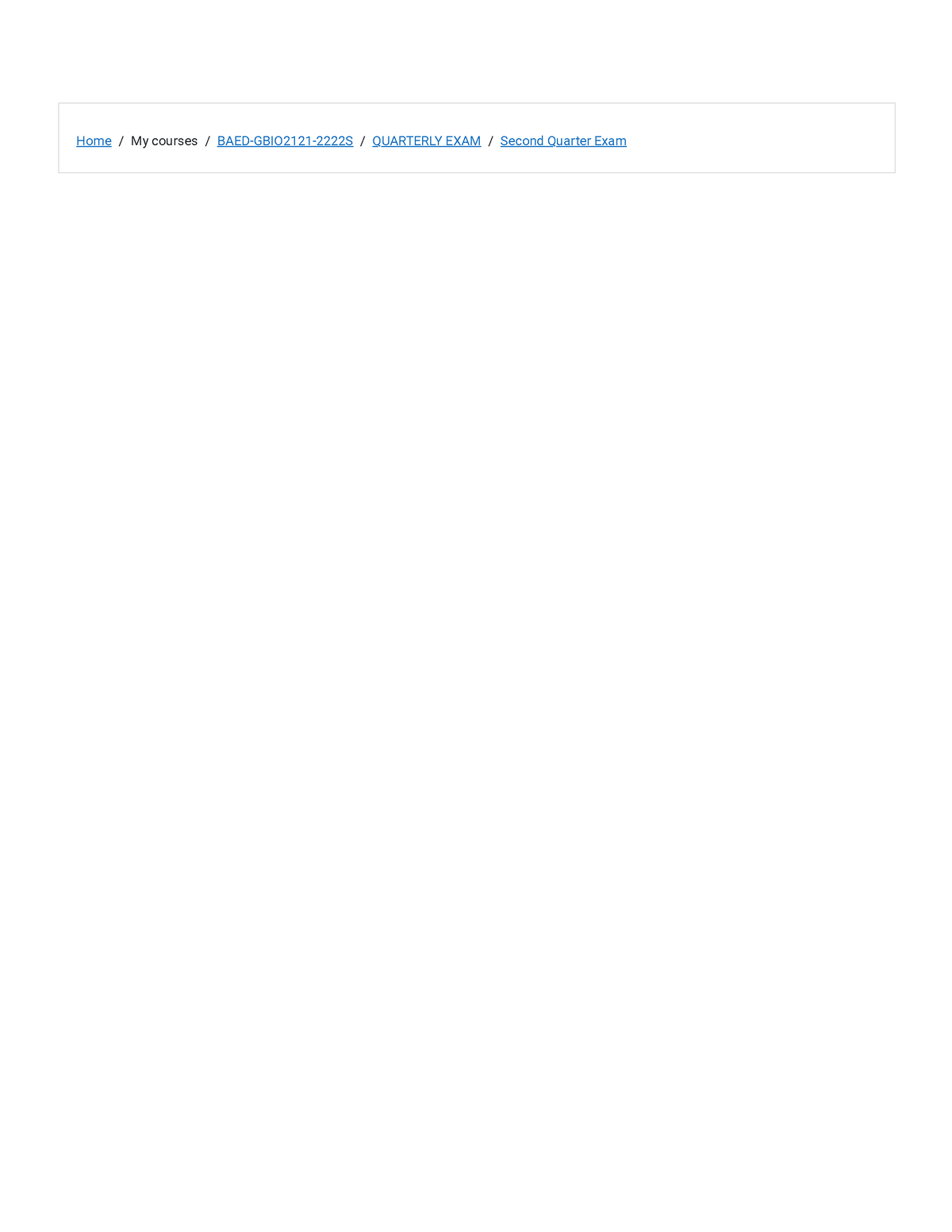This screen capture is from an educational website, likely of a school. The background is predominantly white, featuring a central, empty gray-blue box. Within the box, the following text appears: "Home / My Courses / BAEDGB BIO 2121-222225 / Quarterly Exam / Second Quarter Exam." The text is displayed in shades of blue and black. The box appears to be situated at the bottom of the webpage, as there is no visible content above or below it. Judging by the context, it seems to pertain to a biology course, possibly for a college student. The screen capture focuses solely on this part of the website, with no other courses visible.